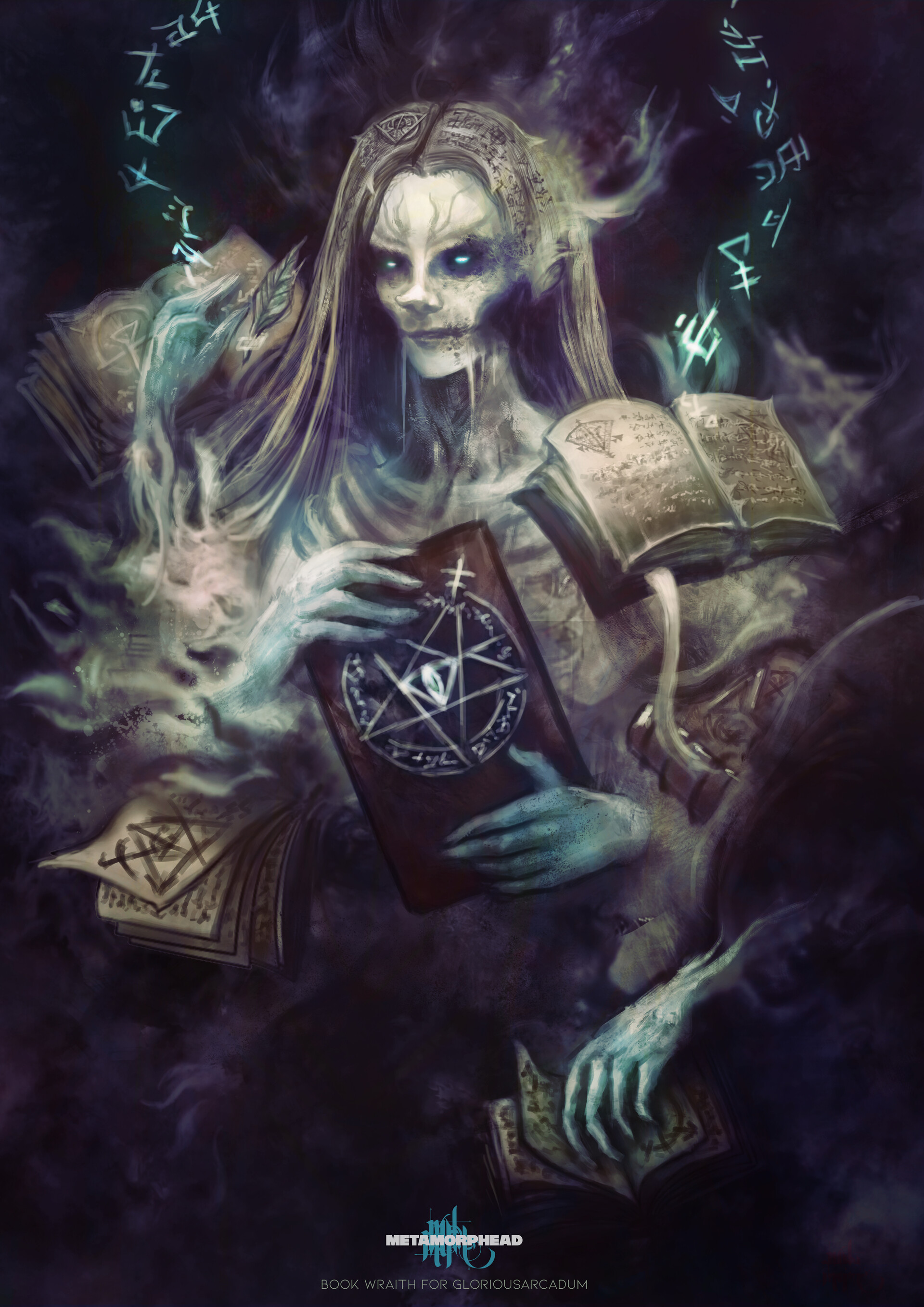In this vertically aligned rectangular poster, the image features a haunting, emaciated female figure with long, stringy light brown hair parted in the middle, juxtaposed against a background of esoteric symbols and books. Her face is strikingly skeletal, marked by visible veins and glowing white eyes that lend an eerie otherworldly presence. Her mouth is closed, albeit slightly distorted.

The figure has four arms, two of which hold a brown leather book adorned with a circular design and a star, possibly a pentagram, suggesting occult themes. One arm rests an open book with gold pages on her left shoulder, while another arm seems to cradle a second book from which pages appear to fly out. Green symbols seem to emanate from some of these books, enhancing the arcane atmosphere.

In the lower right corner, there is an intrusion from another character's hand, also gripping a book. To the right of this spectral woman, near her right side (our left), an image of a snake with symbols emerging from its mouth can be discerned, adding to the mystical and possibly alchemical connotations. The bottom of the poster is emblazoned with text in white all caps, reading "METAMORPH HEAD BOOK WRAITH FOR GLORIOUS ARCADUM," although portions of the text are partially obscured or difficult to decipher.